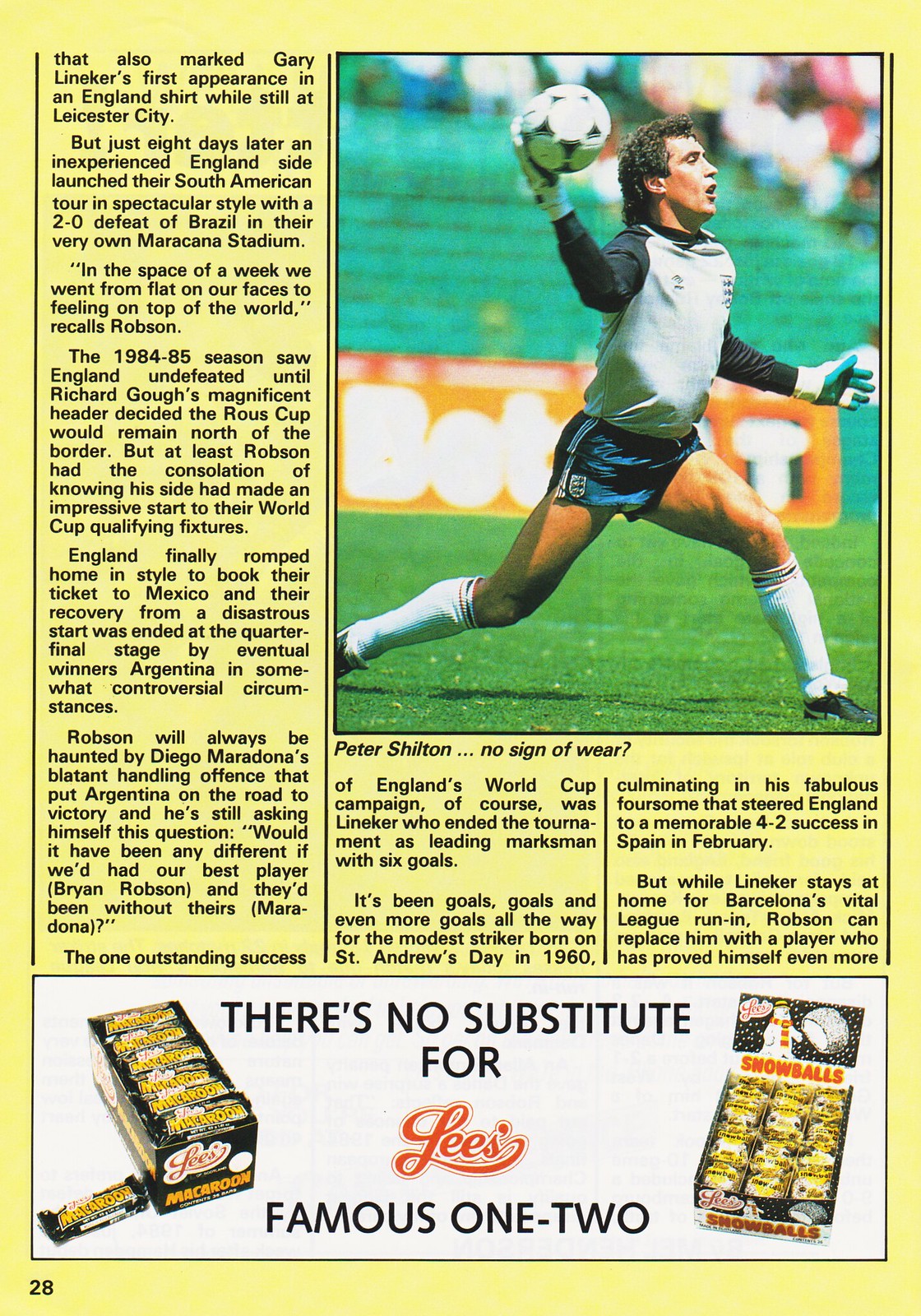This image is a detailed page from a soccer or football publication, specifically page 28. Dominated by a color picture, it features goalkeeper Peter Shilton in action, poised to throw the ball. Shilton is outfitted in blue shorts, a gray and blue top, and white socks that reach up to his knees. Below his image, the caption reads, "Peter Shilton... no sign of wear."

The page also includes an in-depth article discussing significant moments from the 1984-85 season. Highlights include Gary Lineker's debut in the England shirt while still playing for Leicester City and England's 2-0 victory over Brazil at the Maracana Stadium during their South American tour. Additionally, it reflects on England's journey from early setbacks to becoming undefeated until a decisive header by Richard Gow in the Rose Cup.

An advertisement occupies the bottom of the page, promoting Lee's Famous 1-2 treats. The ad showcases a box of macaroons on the left and snowballs on the right, boldly stating, "There's no substitute for Lee's Famous 1-2." The page's background is predominantly yellow and contains detailed scores and information about the soccer season.